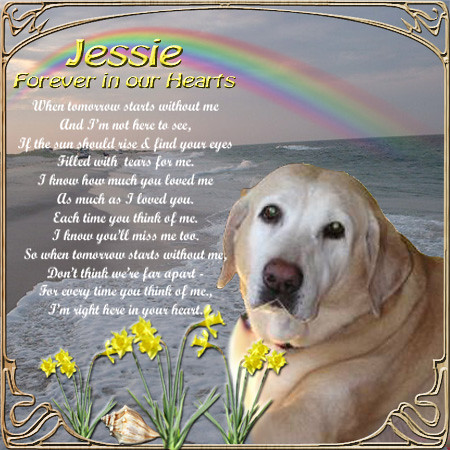The image is a heartfelt memorial for a dog named Jesse, illustrated with a detailed and sentimental composition. Dominating the bottom right corner is Jesse, a tan-colored Labrador with a white face, black eyes, and a brown snout, exuding a gentle presence. Adjacent to Jesse, in the bottom left, lies a tan seashell and a bouquet of delicate yellow flowers with green leaves. Encircling these elements is a golden metallic border that frames the scene elegantly.

In the background, the bottom two-thirds feature a tranquil beach to the left, merging seamlessly into the vibrant blue ocean waves to the right, topped with white foam. Above this serene seaside setting, a colorful rainbow arcs across the sky, adding a touch of hope and beauty to the image.

At the top, in yellow and cursive font, the text tenderly reads: "Jesse, forever in our hearts. When tomorrow starts without me and I'm not here to see, if the sun should rise and find your eyes filled with tears for me. I know how much you loved me, as much as I loved you. Each time you think of me, I know you'll miss me too. So when tomorrow starts without me, don't think we're far apart. For every time you think of me, I'm right here in your heart."

The combination of elements and the poignant poem work together to honor Jesse’s memory, emphasizing the enduring bond between the dog and its loved ones.